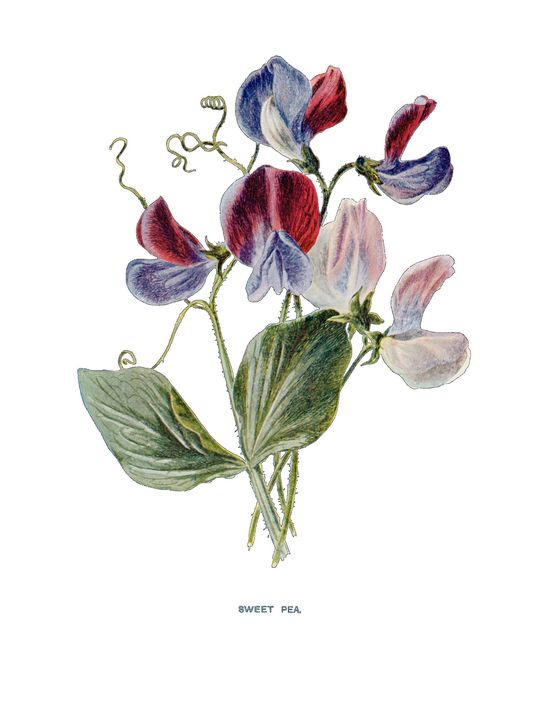This detailed drawing, set against a white background, depicts a "Sweet Pea" flower, labeled in blue letters at the bottom. The intricate illustration showcases six distinct flowers, each emerging from either a pair of large green leaves or slender dark green stems. Notably, one of the stems transitions from a whiter shade at the base to a vibrant green as it ascends.

The diverse petals capture attention with their rich colors and unique formations. Some petals are a striking dark red and blue, with a few combining these hues in an ombre effect from dark blue to red. One central flower exhibits a captivating blend of blue and red petals, while another on the bottom right displays a delicate light pink and blue combination. The delicate beauty of the flowers is further enhanced by swirling green tendrils that curl gracefully off the stems, adding a touch of whimsical elegance to the detailed colored pencil sketch.